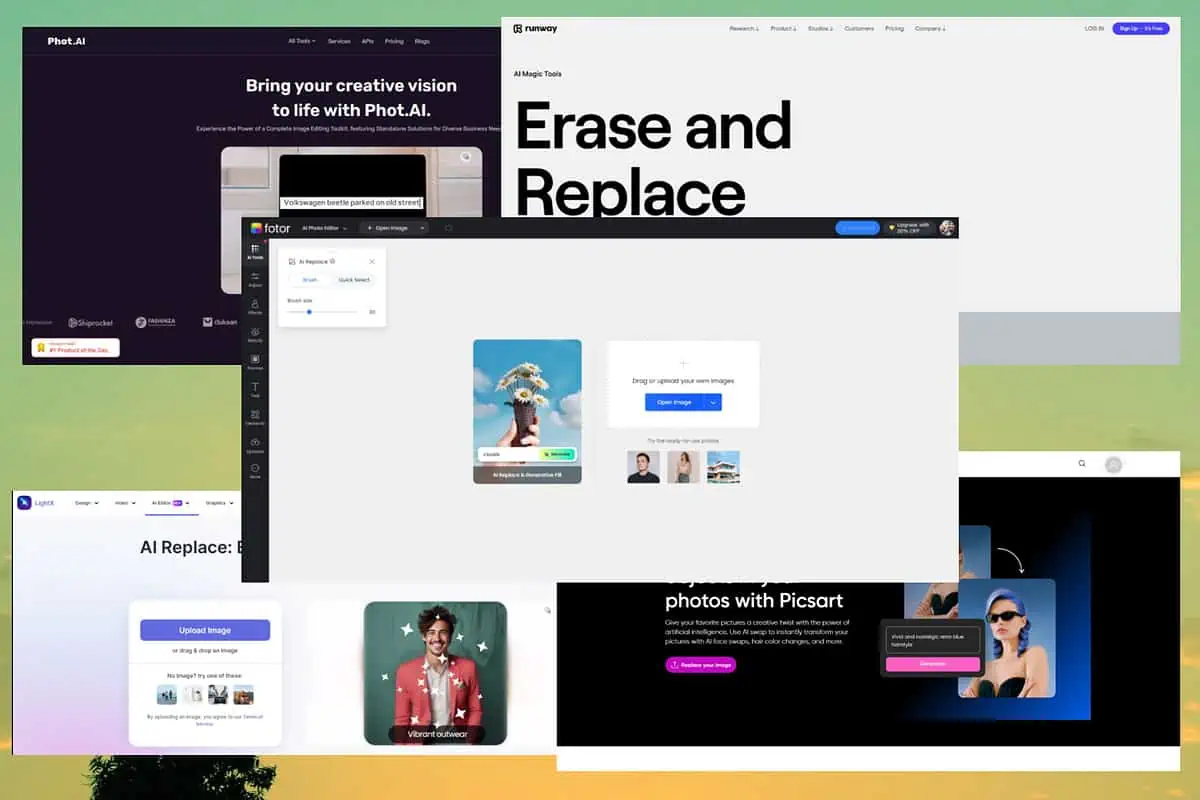In the upper left section of the image, there is a black background window displaying white text that reads "Bring your creative vision to life with PHOT.AI." Adjacent to it is a rounded rectangular frame depicting a partially visible scene resembling white bricks at the bottom and a black area with a white strip at the top. Moving towards the right, there's another window with a white background, featuring an oval in the top right corner, colored dark purple with white text inside. On the left side of this window, the text "Runway" appears in black next to a black logo. Below this, in bold lettering, it says "Erase and Replace."

In the center of the image is an overlay window. To the left center of this overlay, there's a picture of a person holding daisies up towards the sky. On the right side, there is a white rectangle with rounded edges, containing black text and a blue rectangle with white text inside it. At the bottom of this overlay are three different images: one of a male, one of a female, and one resembling a building.

Beneath this central overlay, in the bottom left corner, bold black lettering reads "AI replace:", although part of the text is obscured by the overlay. Additionally, there is a rounded square featuring a purple rectangle with white text. To its right, there is an image of a man with dark hair, a mustache, and a smiling face, surrounded by star-like sparkles.